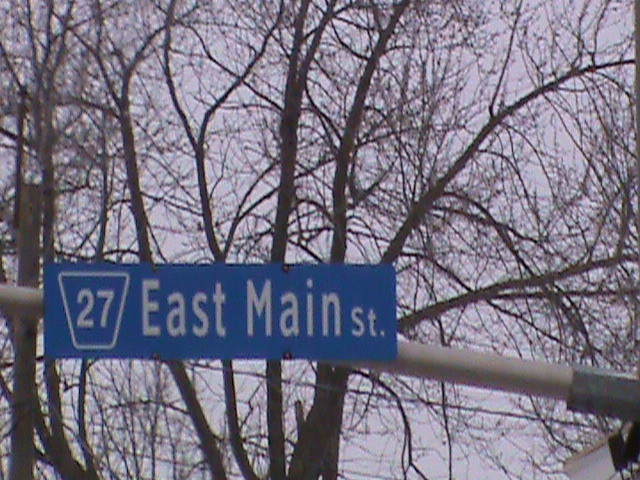This close-up image captures a blue street sign affixed to a horizontal silver metal pole with a dark metal bracket. The sign prominently displays "East Main Street" in white letters, with the number "27" enclosed within a white-bordered rectangular box. The background reveals the stark tops of leafless trees against an overcast gray sky, adding a somber tone to the composition. Just beneath the pole, partially visible, appears to be another structure—possibly a traffic light—adding an element of urban functionality to the scene.